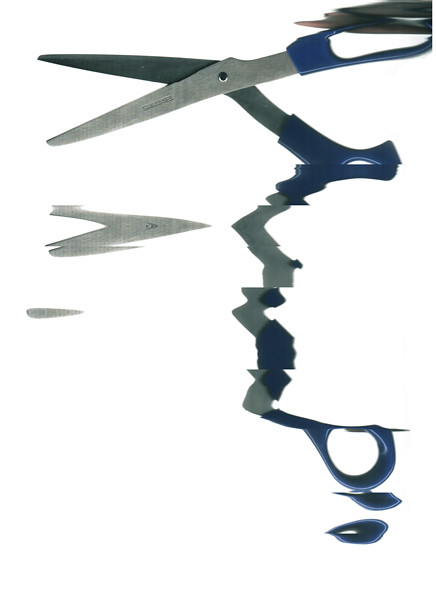The image depicts a pair of scissors with stainless steel blades and blue rubber or plastic grips, positioned on a pure white background. The blades are pointed to the left. Surrounding the scissors, the image features a series of duplicated, zigzagging reflections, creating the illusion of the scissors being partially submerged in water and producing distorted, geometrically patterned replicas both above and below the actual scissors. The reflections, which include parts of the blue handle and metallic blades, appear as if they have been cut and pasted, enhancing the visual effect of a torn or rippled sheet of paper. There is no text present in the image.